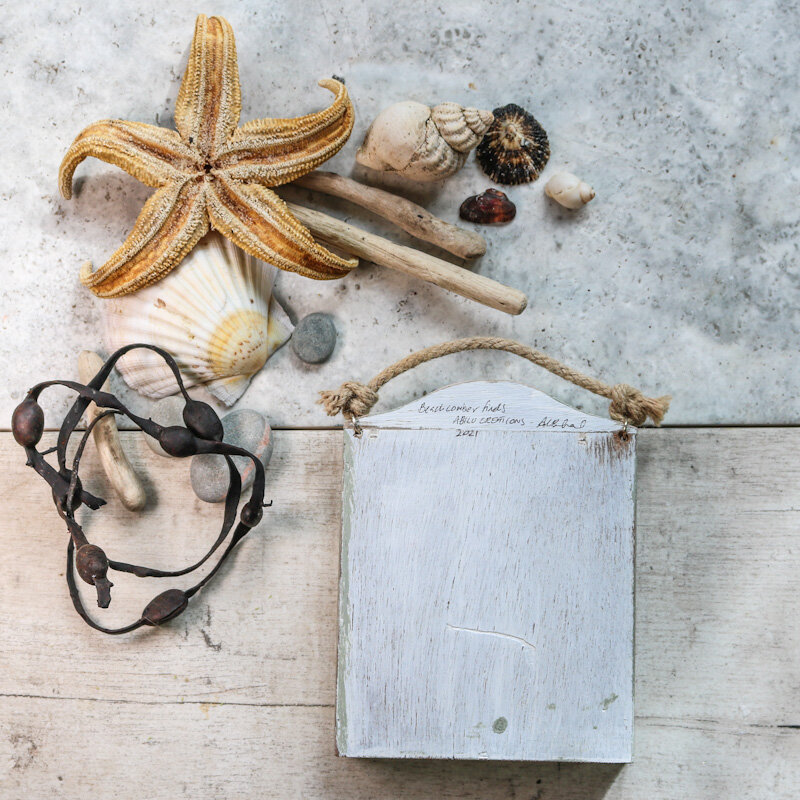In the image, various coastal-themed items are displayed on a surface that transitions from a marble-like texture to a weather-beaten wooden area. At the top, different types of seashells are scattered, including beige and dark brown conch shells, clamshells, and a notable starfish with curled-up legs showcasing its intricate underside. Among the seashells, there are also some ocean rocks in shades of gray, adding to the seaside ambiance.

A black string, potentially leather, decorated with large black beads is placed amid the items. There's also a wooden piece painted white, resembling a sign with an indecipherable cursive inscription at the top. This wooden piece is equipped with a thick rope on either end, suggesting it is meant to be hung. The scene is completed by the presence of sticks and what appears to be driftwood, placing all these objects on a light gray stone and wooden surface, evoking the feeling of a coastal treasure collection.